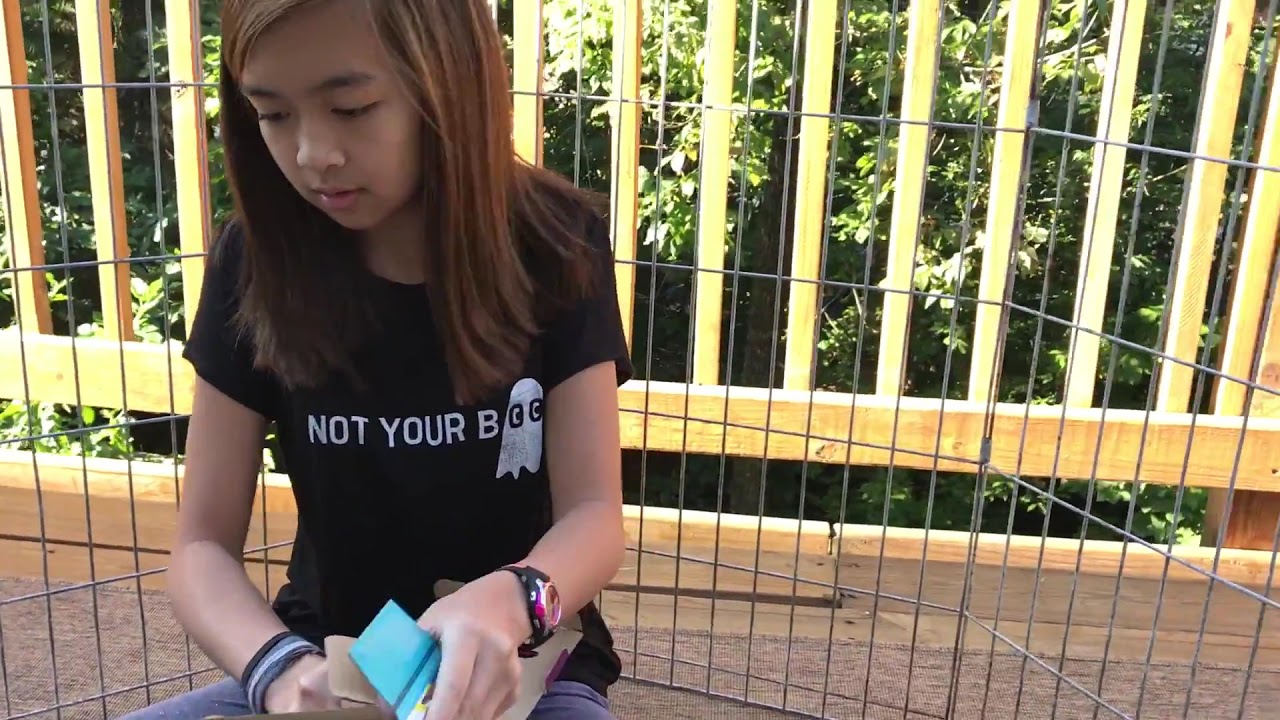A young Asian girl with ombré brown hair — bright at the top and darker towards the bottom — is sitting in front of a metal railing that resembles a cage. She is wearing a black t-shirt with a white graphic that reads "NOT YOUR BOO," where the "O's" form the eyes of a ghost-like image reminiscent of Pac-Man. She has multiple wristbands on her right hand and a pink watch on her left wrist. In her hands, she holds blue paper, possibly a small notebook, and she gazes downward. The setting includes a grayish-brown low pile carpet over wooden planks, and in the background, a yellow wooden fence is partially visible alongside leaves from surrounding trees.